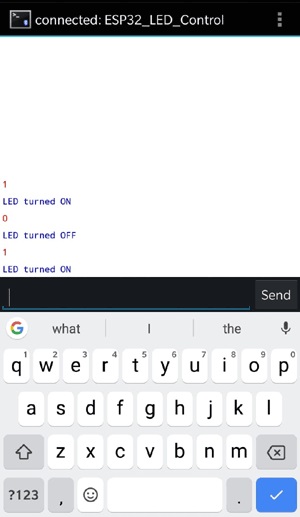In the image, the top section displays a black box containing a small white box. Inside the white box, there's a black and purple symbol resembling an upward-left arrow. The text reads, "Connected ESP32 LED Control," followed by three dots. Below, it states "1: LED turned on" and "0: LED turned off," with "1: LED turned on" repeated once more. Beneath this, there's another black box with a thin white line on the left and the word "Send" on the right.

The lower section of the image features a keyboard with a purple background. On the top row of the keyboard, there is a white circle with the multicolored Google "G" (red, yellow, blue, and green). To the right of the "G," various icons and text are visible, including a microphone symbol. The main keyboard comprises white keys with black lettering.

On the lower row, there is a purple button with an upward arrow, a purple button with a question mark, and a key labeled "1 2 3." To the right, you'll find a small box with a comma and another small white box with a smiley face. Further right, there is a purple box with a period and a purple box with a square containing an "X." Finally, on the far right, a blue box with a checkmark completes the layout.